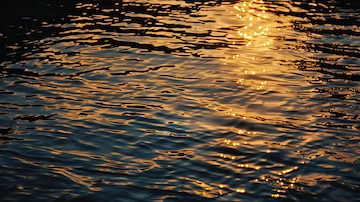This high-quality photograph captures the surface of a large body of water, possibly a lake, at either sunrise or sunset. The image is taken at a close angle to the water, emphasizing the subtle movements and slight ripples across its dark surface. The water appears deep blue and almost black towards the bottom and corners of the image. As the eye moves upward and towards the center, the color transitions to a lighter purple punctuated by bright, streaking reflections of yellow sunlight. The upper left corner of the image remains shadowy and dark, compared to the upper right corner which is bathed in more vibrant yellow beams and streaks of purple and black. The image is devoid of text and other objects, focusing solely on the interplay between light and water.